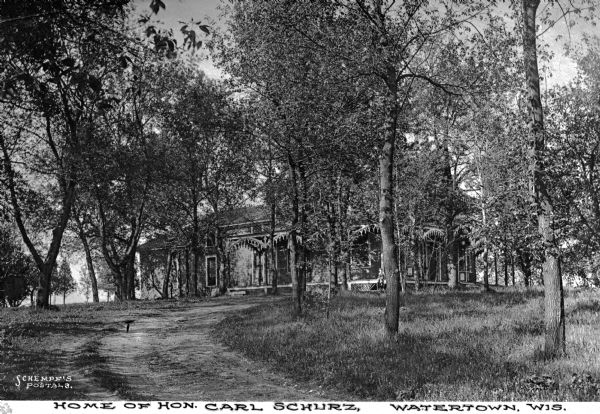This horizontally aligned rectangular black-and-white photograph, possibly an old photograph rather than a pencil drawing, features a grand house in the far background with numerous windows. The sky above the house appears a bit cloudy and bright. A curved dirt pathway starts from the bottom front of the image, leading up to the house. On either side of the pathway, there is grass and numerous tall trees with slender trunks and abundant leaves. White text in the bottom left-hand corner reads "Shemps Postals." Beneath the photograph, in black text, it states, "Home of HON. Carl Schurz, Watertown, Wisconsin," indicating the residence of the Honorable Carl Schurz situated in Watertown, Wisconsin.